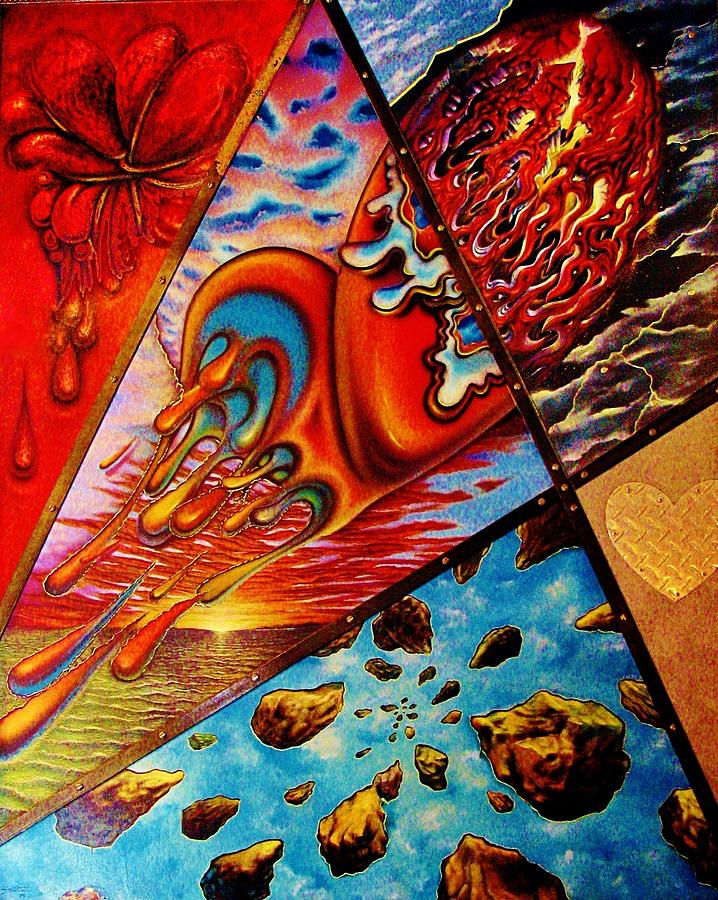The image presents an intricate piece of abstract artwork, divided into segments by intersecting black lines and joined by small silver finishes, possibly nails or screws. Each segment showcases a distinct scene, employing a vivid palette of blues, reds, oranges, and yellows. In the upper left corner, a predominantly red picture displays a flower dripping blood, creating a stark and striking visual. Just below and to the right of this, a surreal skyline emerges, featuring a heart-like object that appears to melt and drip into a sunset over the ocean. Moving to the upper right corner, a flesh-like, torn texture with yellow tones is seen, framed by a blue sky with hints of purple lightning. Below this, a panel featuring a copper hue portrays a heart bleeding or melting. The bottom section is dominated by an aqua blue void accented with white splotches, from which large teardrop-shaped or asteroid-like boulders seem to fall. This complex, multi-faceted artwork leaves a lasting impression with its detailed and diverse elements.